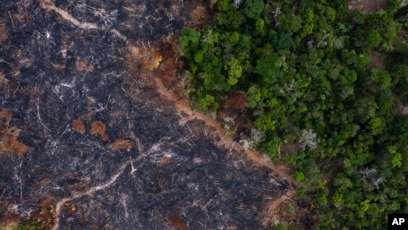This image is an aerial photograph showing a detailed yet slightly out-of-focus view of a landscape divided into distinct regions. The right side is dominated by a thick, verdant forest, with shades of bright and lush green suggesting a dense canopy. Adjacent to this forested area, on the left side, is a darker region, possibly indicative of a terrain affected by a forest fire, contributing to the predominant dark hues. Tiny, winding roads meander through both regions with one notable road stretching from the upper left into the forest and another crossing diagonally from the lower left. Additionally, patches of pinkish and purple hues are scattered across the image, hinting at variations in land or possibly geological fault lines. Despite the photograph's small size, some text appears in white on the lower right, reading "AP." The point of view is high above, creating a map-like perspective of the landscape below.